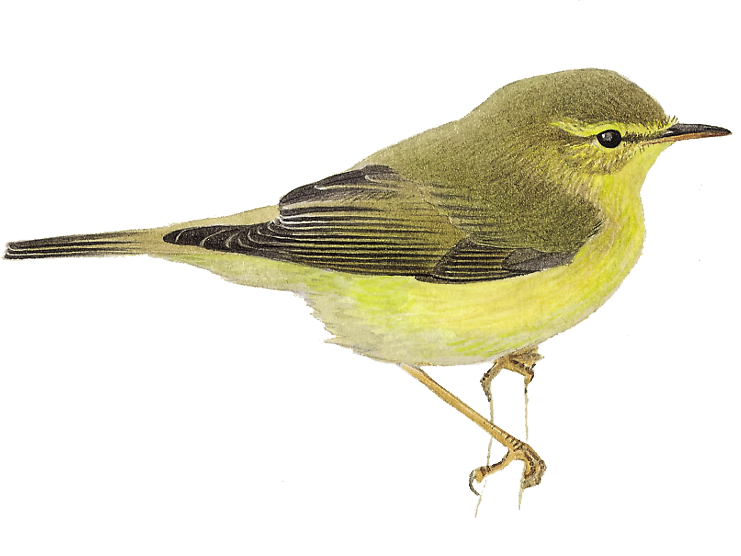This image showcases a realistic drawing or digital rendering of a small bird, possibly a sparrow or chickadee, set against a pure white background. The bird is perched on a vertically oriented branch, displaying its intricate details. It is facing to the right, allowing a clear view of its features. 

The bird's body is predominantly yellow with a greenish tinge, particularly on its breast and underside. Its head is mostly dark gray to black with interspersed yellow-green hues. The dark, reflective eyes add a lifelike quality to the depiction. 

The beak is distinctive with its black upper part and orange lower part. The wings, stretching back along its body, are primarily black interspersed with yellow-green stripes. The tail shares a similar black and yellow-green striped pattern. The legs of the bird are long and a mix of yellowish and brown tones, with talons featuring dark lines and spots. Overall, the bird presents a vivid spectrum of green, black, and yellow across its body, wings, and tail.